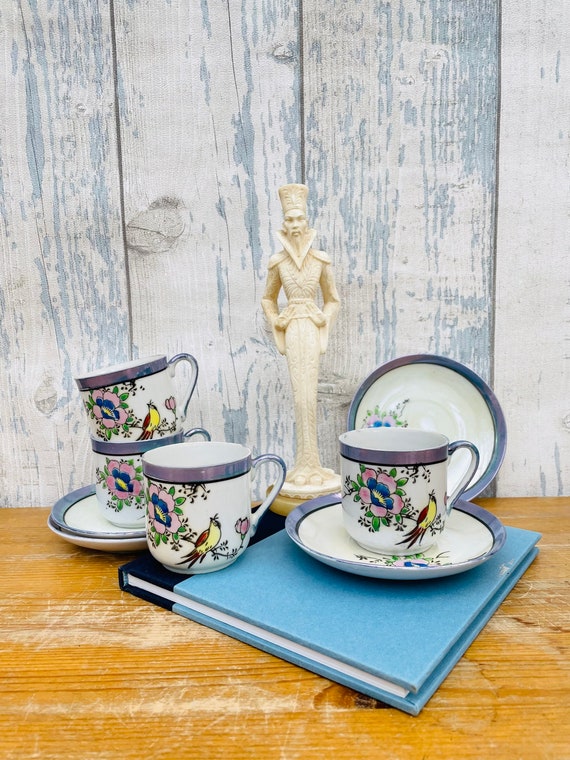The image depicts a detailed setting on a brown wooden counter, complemented by a grayish or whitish wooden backdrop. Central to the scene is a closed book with a light blue and dark blue cover, lying flat on the counter. Resting atop the book are two ornate white teacups, each adorned with lavender flowers featuring blue and yellow centers, accompanied by green leaves and a bird painted in yellow and red hues. These teacups have silver-rimmed lips and are paired with saucers that also bear matching floral designs and silver perimeters. 

Additionally, a small, intricately crafted statue made of an ivory or off-white material stands amongst the teacups. The statue, approximately 10 inches tall, is modeled as a thin figure clad in robes and wearing a distinctive round hat with a flat top. To the left, another pair of similarly designed teacups rest on their saucers, completing the elegant and artistic composition of the scene.